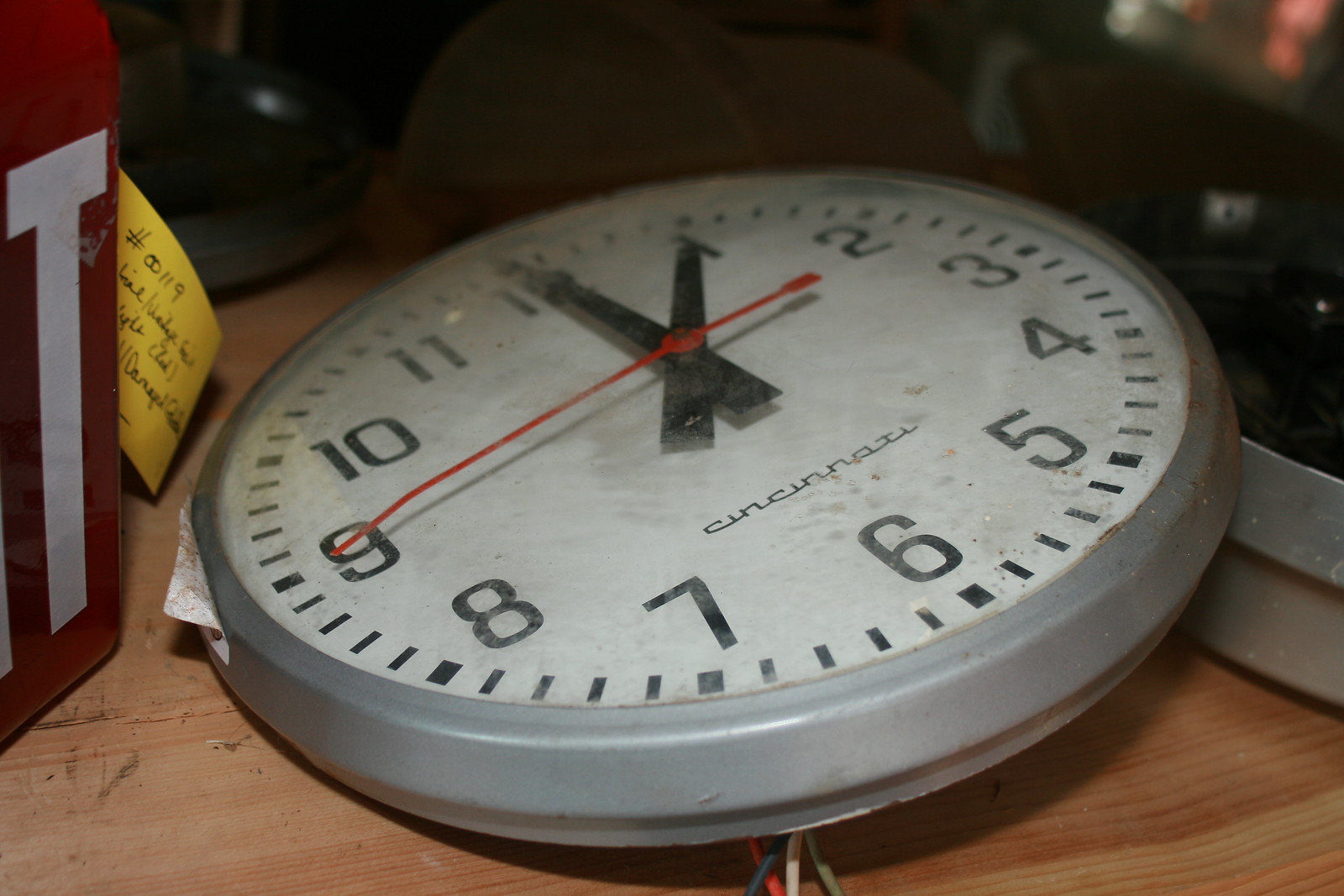This color photograph captures a close-up of an old, gray metal clock lying on its side on a light wooden base, likely in a repair shop. The round clock, showing noticeable signs of deterioration with a dirty, dusty crystal and rust on its housing, has a white face with black numbers and black hands indicating one o'clock, while its red second hand points to the nine. The clock, marked "Cincinnati" above the number six, appears disconnected, evidenced by loose wires extending from beneath it near the seven. The cluttered background reveals a brown box with a white 'T' and a yellow tag labeled '0019,' and the clock is propped against another metal object, possibly another clock, adding to the sense of disarray.